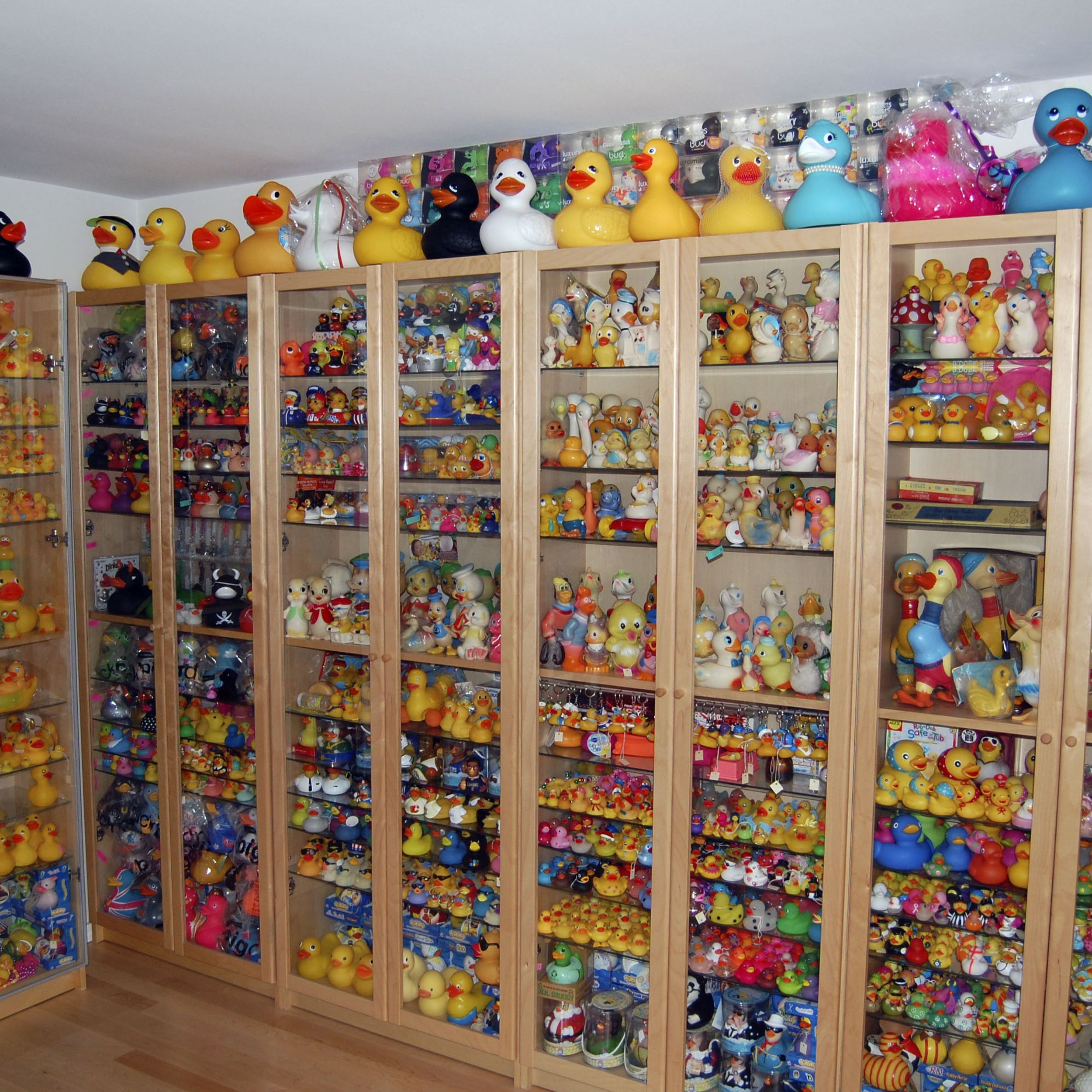A mesmerizing collection of toy ducks is showcased within a series of five glass-paneled cabinets, each with two doors, proudly displaying a breathtaking array of colorful and varied ducks. Each cabinet contains ten shelves, meticulously organized and brimming with ducks of all shapes and sizes. The majority of the ducks are classic yellow with orange bills, but the collection also boasts an impressive diversity, including ducks in white, black, blue, pink, purple, and green, with some decorated in festive wear or different outfits like sunglasses, handkerchiefs, and even Christmas attire. The ducks range from antique to modern, some exhibiting distinct patterns and joyful expressions. Atop the cabinets, larger ducks that couldn't fit inside perch brilliantly, adding to the vibrant display with their own array of colors including blue, pink, and black. This animated and cheerful room pulsates with the engaging sight of this extensive and joyful duck collection, reflecting a lifetimes' dedication and diverse acquisitions from various places and eras.